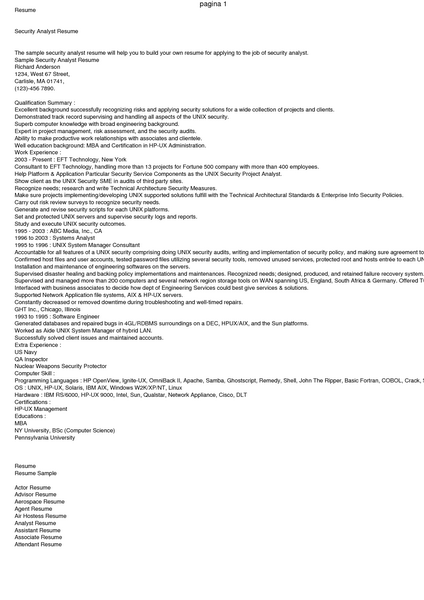The image, originating from an online application, showcases a segment of a resume against a stark white background. At the top left corner, the resume is labeled with the heading "Resume," rendered in black text. Centered at the top, the document bears the name "Pagina 1." The entire content of the resume is meticulously left-justified, ensuring that all text aligns seamlessly with the left margin.

Directly beneath the word "Resume," the title "Security Analyst Resume" is prominently displayed. Following this title, the resume comprises the address of the owner, succeeded by a space. The subsequent section is a comprehensive "Qualification Summary," detailing the owner's qualifications and professional experiences. This summary culminates with the mention of "Pennsylvania University."

The remainder of the resume continues with additional sections, each containing pertinent information about the resume owner’s credentials and background.